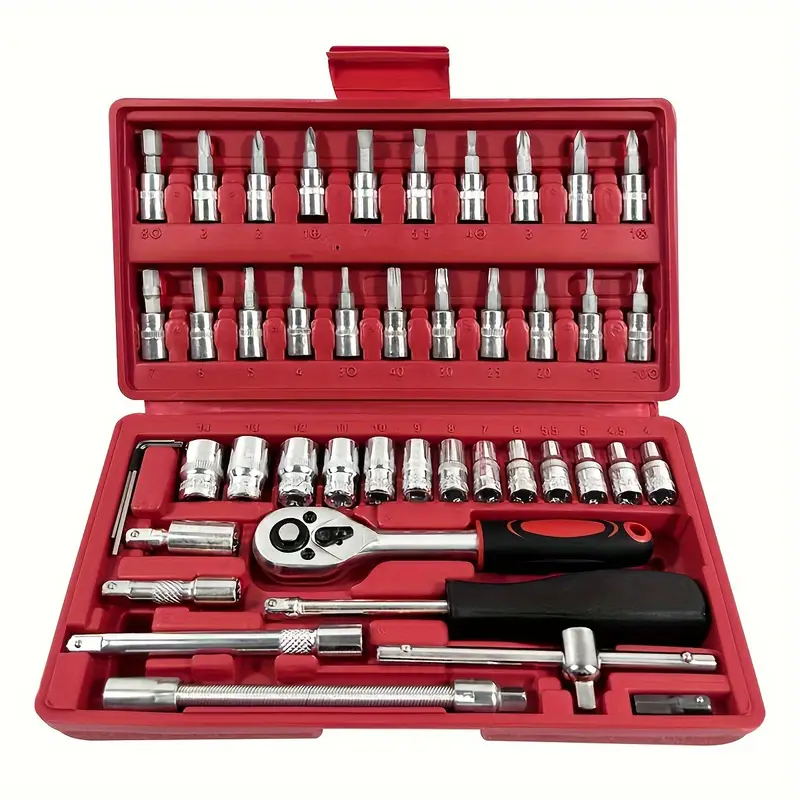The image depicts a detailed tool set housed in a red plastic carrying case that is currently open, revealing its contents. The top section of the case holds approximately 20 diverse screwdriver bits, arranged in two neat rows, each designed to accommodate different screw types, shapes, and sizes. Just below, the bottom section is organized with four rows of socket wrenches and tubular extenders, crafted from silver metal. The foremost row in this section contains various sizes of sockets, likely labeled with numeric size indicators that are somewhat obscured in the image. Central to the bottom compartment is a socket wrench with distinctive black handles, along with multiple extensions, intended to provide extra length for reaching challenging areas. This comprehensive tool set is both colorful and multifunctional, equipped for numerous tasks involving various bolt and screw sizes.